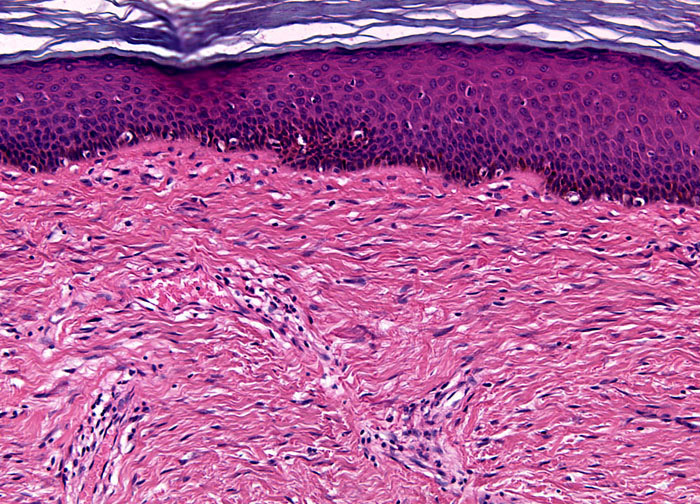The image is a detailed, abstract painting that appears to depict a cross-section of a membrane or cellular structure. The artwork predominantly features shades of purple, with areas of red and pink, and exhibits a layered composition. The bottom section is a light purple that flows in long, extended strands with darker purple dots interspersed. Above this is a darker, more solid-looking purple layer comprised of small, tightly packed circular patterns. The topmost section combines purple and white in almost striped formations, interlaced with black vein-like lines and dots, evoking the structure of a blood vessel. The painting has an asymmetrical, oceanic wave-like movement, enhanced by swirling patterns and white highlights that dance across the foreground and background. This intricate interplay of colors and structures creates a vibrant, dynamic visual reminiscent of microscopic life forms and fluid environments.